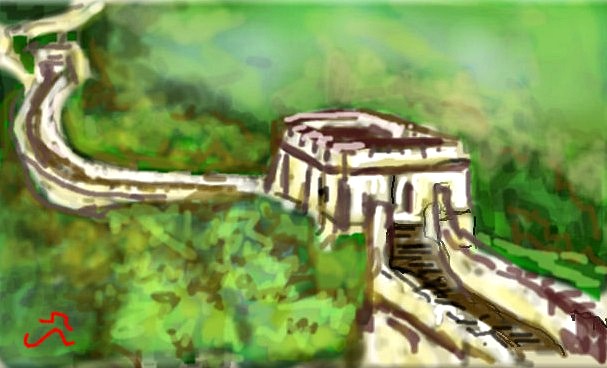This is a rich watercolor illustration depicting a panoramic view of a historic structure, resembling the Great Wall of China, surrounded by lush greenery. The predominant colors are green hues for the trees and low-lying vegetation, and there are slivers of blue smudged into the sky. At the center of the image is a large, tan-colored building with brown outlines, likely an ornate castle-like structure or a fortification. An off-white pathway with a dark brown center winds through the landscape, wrapping around a sizable hill and suggesting an old, well-trodden route. 

In the foreground, we see a covered bridge, almost tunnel-like, characterized by off-white walls, dark windows, and a black top, with a white vehicle traversing through it. This pathway extends to become the grand Great Wall, rendered in shades of tan for the bricks and dark brown for the walkway, curling majestically towards the left and continuing downward through the front of the painting. This immense structure is flanked by forested areas painted in variegated greens and dark yellows, mixed with some accents of brown, enhancing the natural, verdant surroundings. 

In the bottom left corner, a small, enigmatic sign composed of a few line-like symbols, possibly the artist's signature, is present. Notably, the scene is devoid of people, capturing a serene, almost timeless quality.